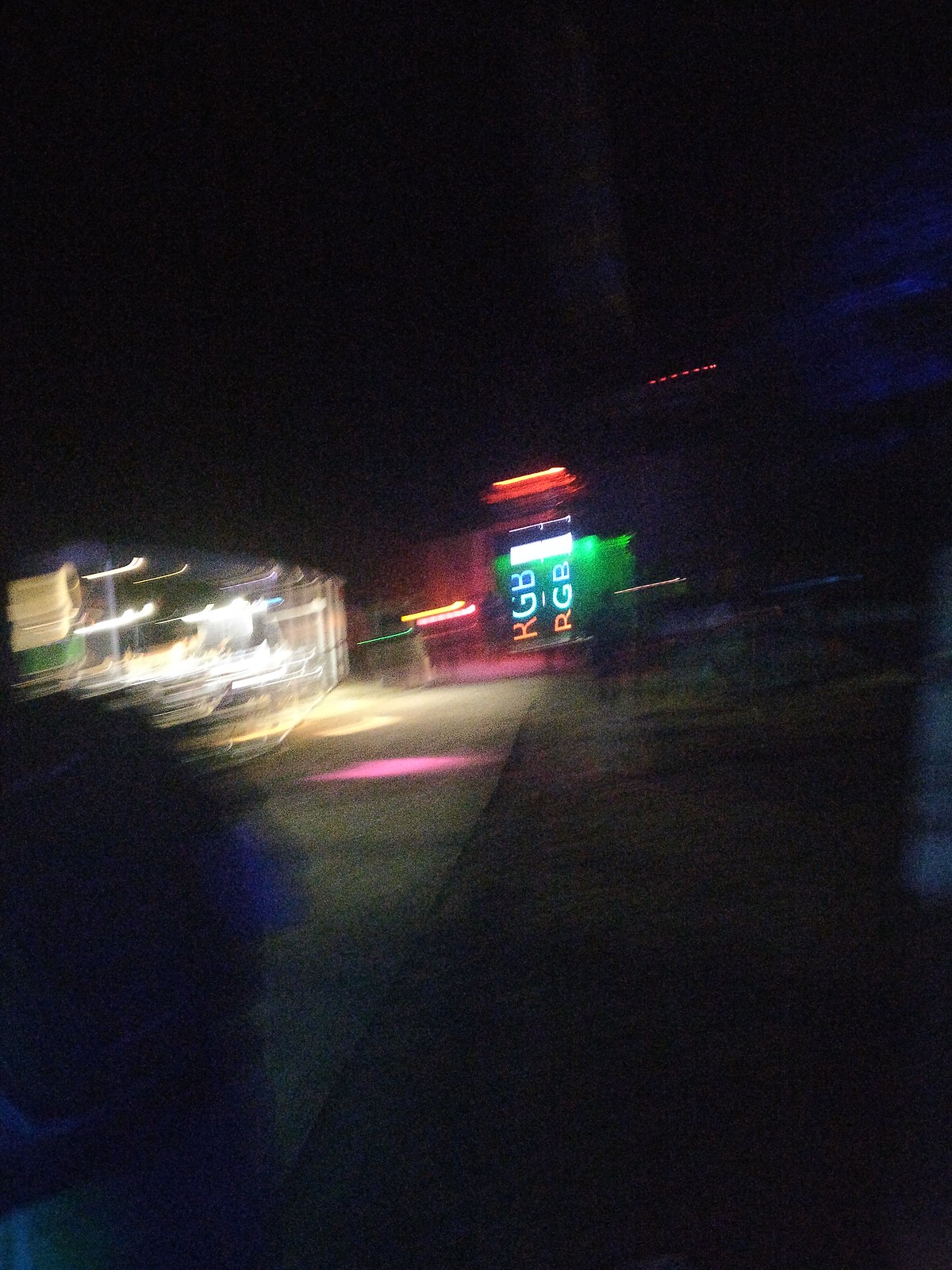This photograph, though blurry and seemingly taken from a moving car, captures the entranceway of what appears to be a nightclub or business establishment. The image shows two prominent doors, each adorned with the letters "RGB" in bold capital letters. Above the door on the right, a line of small red lights flickers, casting a faint glow. Neon lights frame both sides of the entrance, adding a vibrant ambiance. To the left of the doorway, a canopy extends outward, with fluorescent lights illuminating its underside. A nearby object with a yellowish top and green base, likely a vehicle, is visible on the left side of the image. The ground in front of the door reflects a mix of pink and yellow light, enhancing the colorful scene. The foreground of the photo is marked by a shadowy blur, suggesting it was shot from within a moving vehicle, adding to the dynamic feel of the scene.